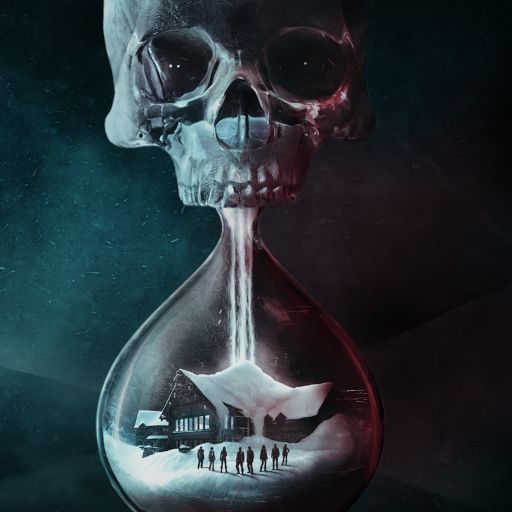The image depicts an abstract, graphic rendition of an hourglass. The upper portion of the hourglass seamlessly transforms into the upper segment of a human skull, which lacks the jawbone. The skull, colored in shades of gray, features clearly detailed eye sockets, nose cavity, and upper teeth. Snow pours from the skull's teeth like sand in a traditional hourglass, cascading down into the bottom half where an intricate winter scene emerges. This scene includes a house with a snow-covered roof, surrounded by snow-laden ground. Outside the house, eight indistinct figures form a V-shape, seemingly observing the accumulating snow. The artwork merges the macabre and the serene, juxtaposing the inevitability of time with the peaceful quiet of a snowy landscape.